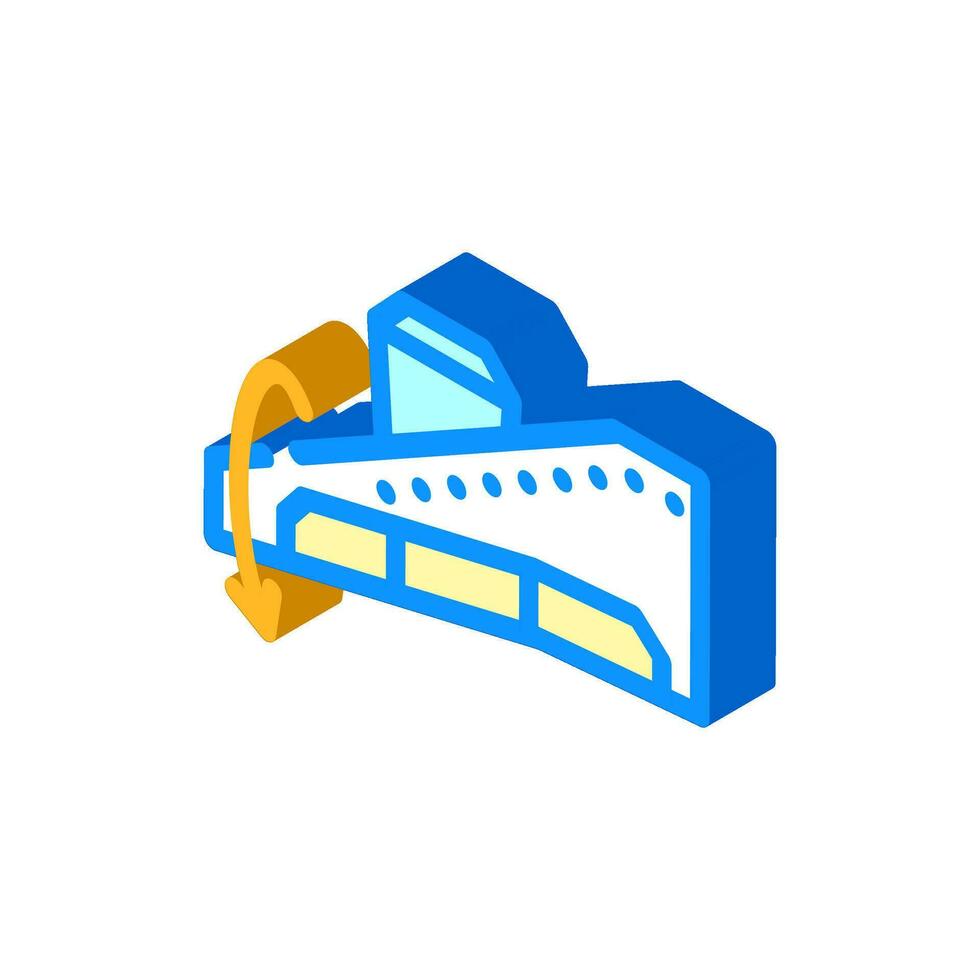The image is a detailed vector-style illustration set against a white background, resembling an icon typically used for applications or mobile apps. Central to the image is a blue and white structure shaped like an escalator or a bobsled, rendered in a 3D style with a blue outline and darker blue edges giving it depth. The structure has multiple blue circles or dots along its side. A prominent yellow arrow starts at the top of the icon, curving downward in a smooth motion. The image also features a yellow section resembling a railing, adding to the visual complexity of the icon. Overall, the illustration's clean white background emphasizes the vibrant blue and yellow elements, creating a visually engaging and detailed design.